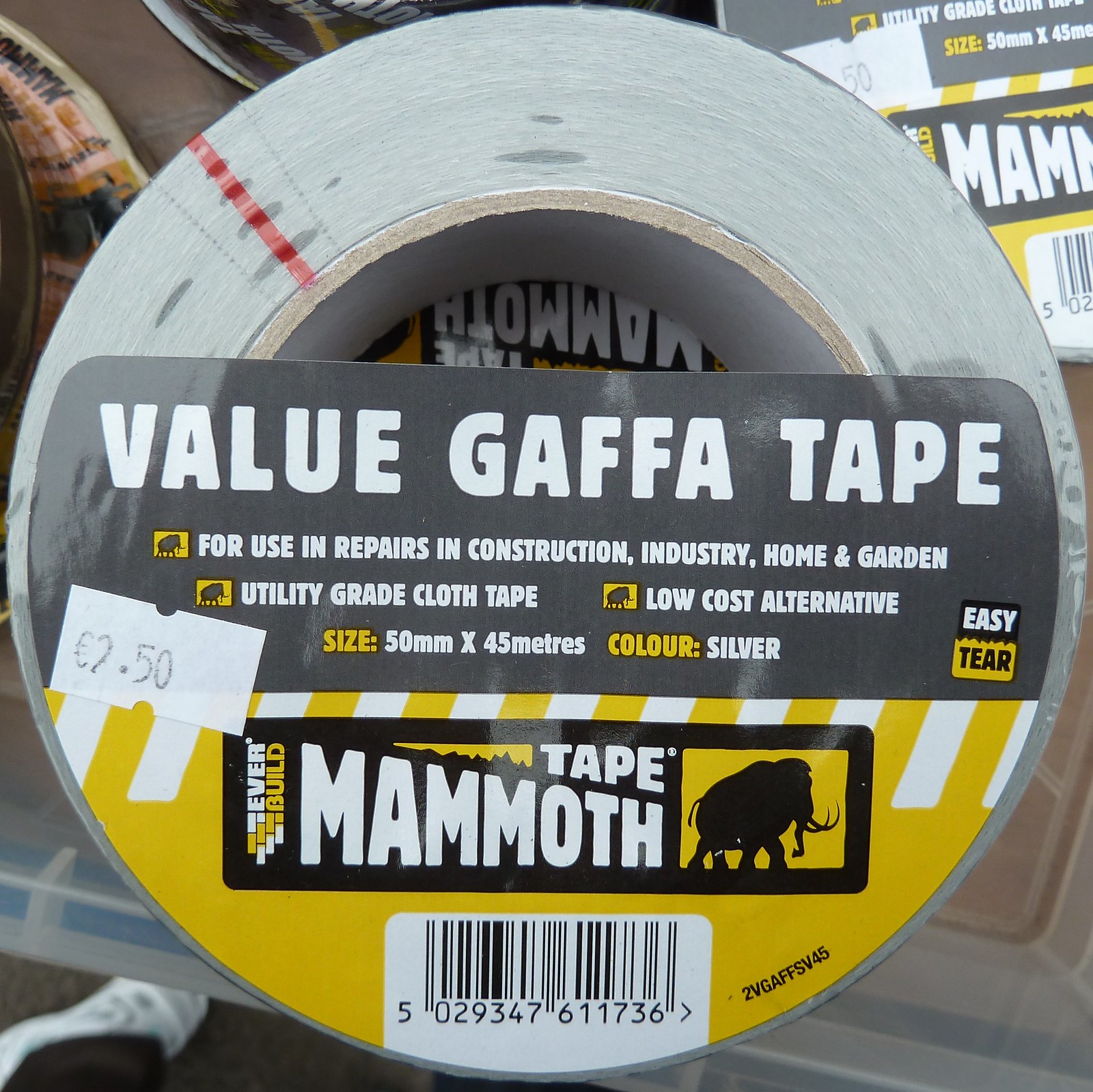The image displays a brand new roll of Value Gaffa Tape, resembling duct tape. The tape is viewed from the side, showcasing its silver color and the comprehensive label wrapped around it. The label is predominantly yellow with white stripes and contains detailed white text, including "Value Gaffa Tape for use in repairs and construction, industry, home and garden, utility grade cloth tape, low cost alternative, 50mm x 45m, color silver, easy tear." The logo features the silhouette of a mammoth with long tusks walking toward the right. Beneath the logo is a scannable barcode and a price tag of $2.50. The packaging is enclosed in plastic, and a portion of a man's foot, wearing what might be a Converse sneaker or slipper, is visible beneath the roll.